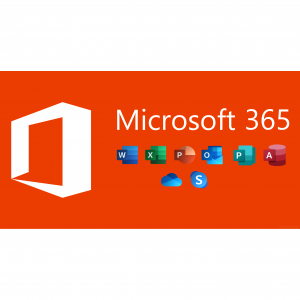The image is a rectangular logo, typically seen on signage representing a product or business. The backdrop of the logo is an orange-red gradient. On the left side of the image, there is a white icon resembling a tower PC. To the right of this icon, the text "Microsoft 365" is prominently displayed. Below the text, there is a sequence of distinct icons, each enclosed in its own square or circle:

- A blue square featuring a white "W"
- A green square containing a white "X"
- A circular icon with a white "P"
- An envelope-shaped blue icon with a white "O"
- Another green icon with a white "P"
- A cylindrical style "A" 
- A cloud icon
- Finally, a blue "S" with a corresponding bluish icon beneath it

These icons represent various applications and services within the Microsoft 365 suite.